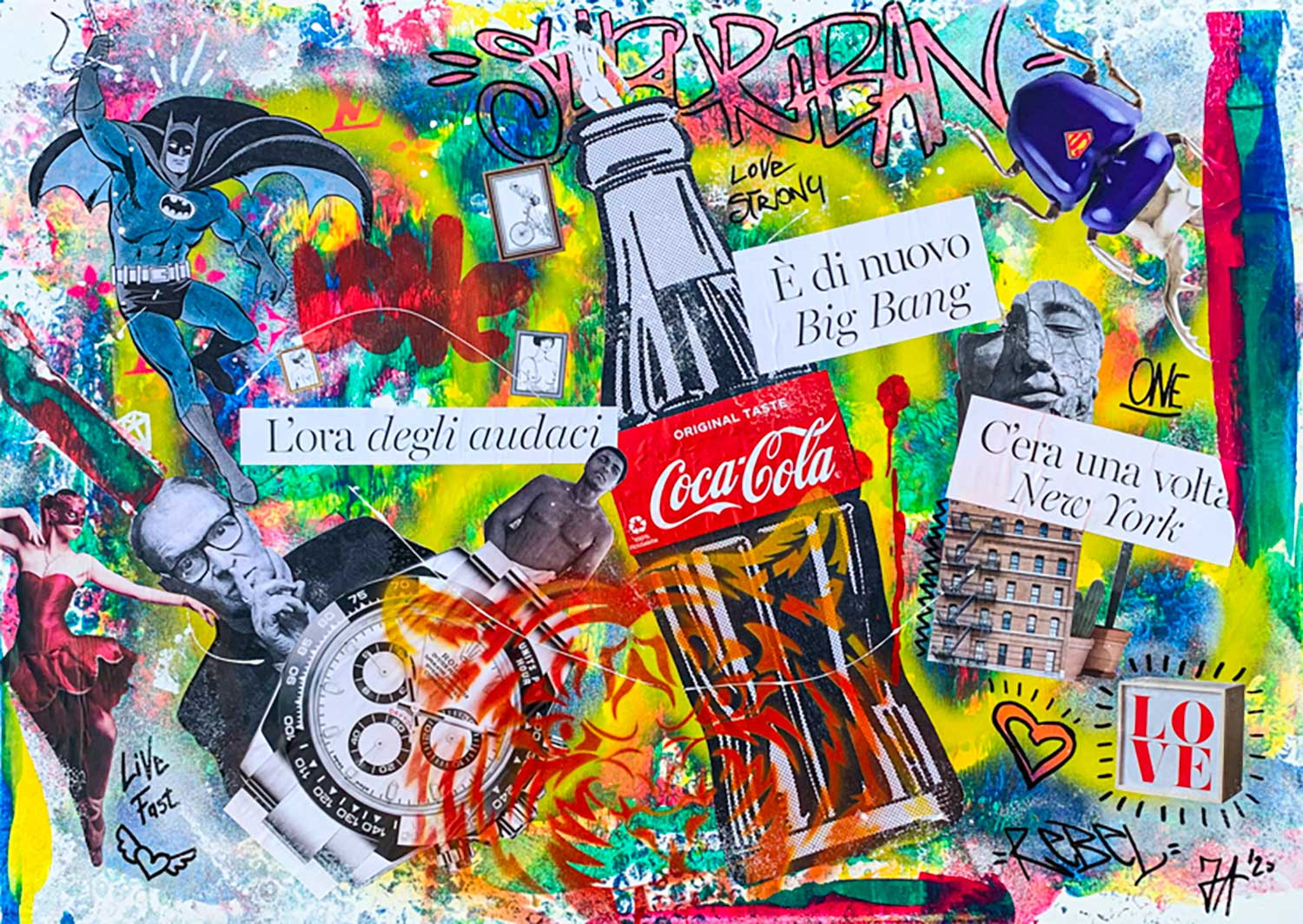The poster image portrays an intricate mural-like collage that melds vibrant graphic art with a plethora of distinct elements. Dominating the background are richly colored areas, featuring prominent hues of green and yellow, alongside with a rainbow coloring scheme. At the upper left corner, Batman is depicted flying, providing a dynamic contrast to the otherwise static graphic elements. In the center, a Coca-Cola bottle prominently displays the brand’s name, encapsulated within the vibrant chaos of surrounding details.

Interspersed within the collage, several figures and symbols demand attention. A man with his eyes closed and a wristwatch can be noticed, and another man holds a finger to his mouth, hinting at Freemason symbolism. Text elements such as "Big Bang", "New York", and names like "Lourdes Aguilera", "Evie Nova", and "Serra Luna" are scattered throughout, each adding to the narrative complexity. The word "love" and a heart symbol offer a softer element to the collage, juxtaposing the more intense aspects.

In the upper right part of the image, an upside-down Superman symbol is positioned, contributing to the layer of pop culture references embedded within the mural. A building emerges from the collage, subtly anchoring the scene amidst the graphic interplay of colors and symbols. This organized style of graffiti creates a visually cohesive yet chaotic display that captures the viewer's attention with its layered storytelling and artistic vibrancy.